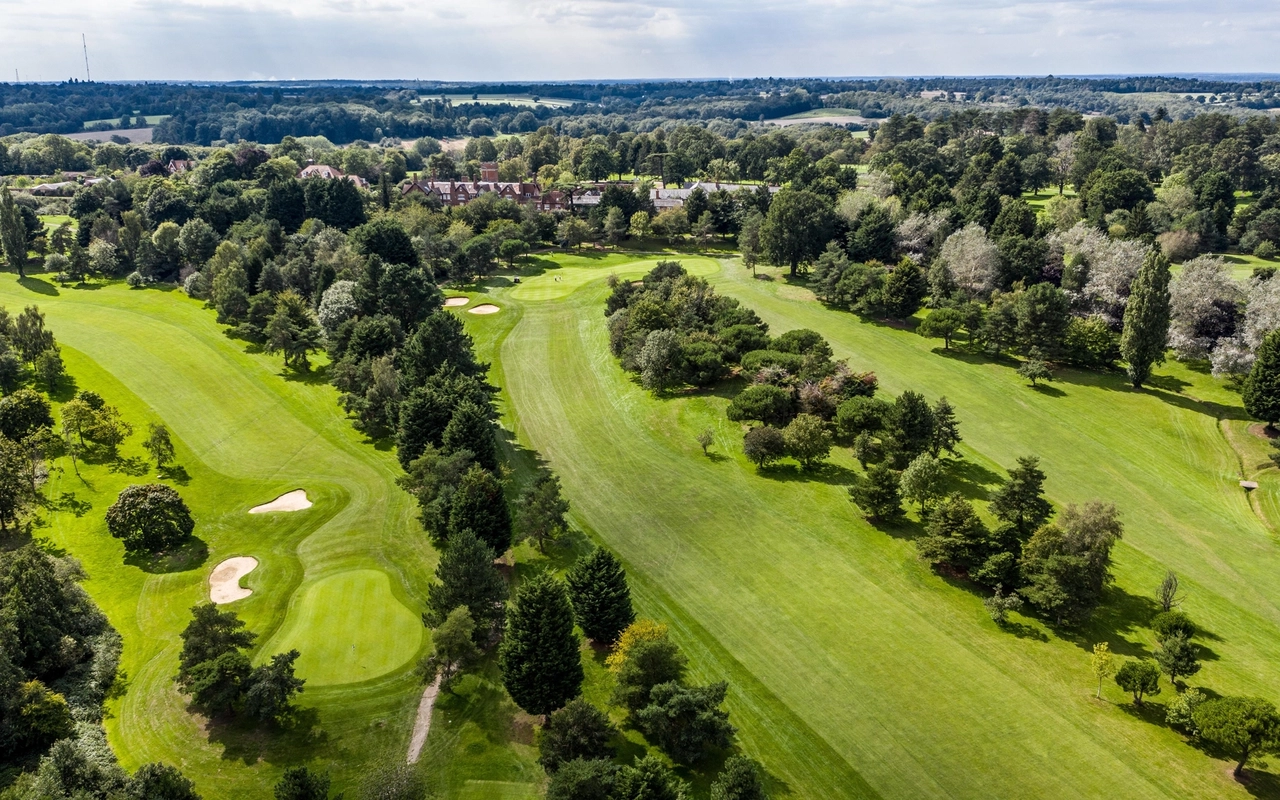This aerial photograph captures an extensive view of a golf course landscape under a partly cloudy, medium blue sky. The image prominently features three fairways, each lined with trees of varying shades—medium green, dark green, and silvery gray. The left fairway includes a putting green and two adjacent sand traps, transitioning to yellowish-green grass. Another fairway in the center of the image also displays two sand traps to the left of a large green, while a third fairway runs to the right, separated by rows of trees. Towards the upper third of the image, a large red-brick clubhouse or manor is surrounded by more trees, with distant rooftops of multi-story buildings in a mix of brown, red, and white. In the far background, additional fields and trees are visible, and there is a faint outline of a radio tower. The scene is well-lit by daylight, with a hint of possible rain far off in the distance.